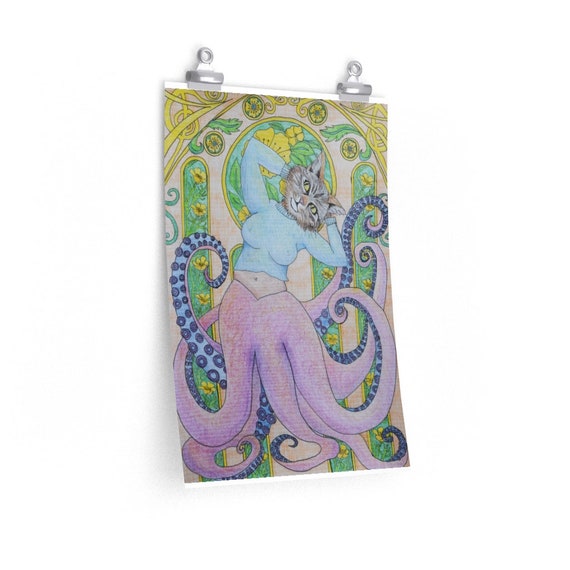This image showcases a unique and whimsical Art Nouveau drawing, expertly displayed on a white wall using two clips attached to brackets. The subject is an imaginative creature with the head of a gray and brown cat, adorned with big ears, and displaying a playful, slightly tilted expression. The cat's head crowns the torso and arms of a woman, who is dressed in a cropped blue shirt that subtly reveals her belly. The lower half of this fantastical being transitions into the tentacles of an octopus, with the top side of the tentacles a light purple-pink and the underside featuring blue suckers.

The background of the drawing is an intricate pattern of gold, red, and green, interspersed with delicate floral designs, creating a vibrant and enchanting setting. The overall aesthetic of the drawing is very much in the Art Nouveau style, combining natural forms and elegant lines to produce a truly captivating and fanciful piece of art.